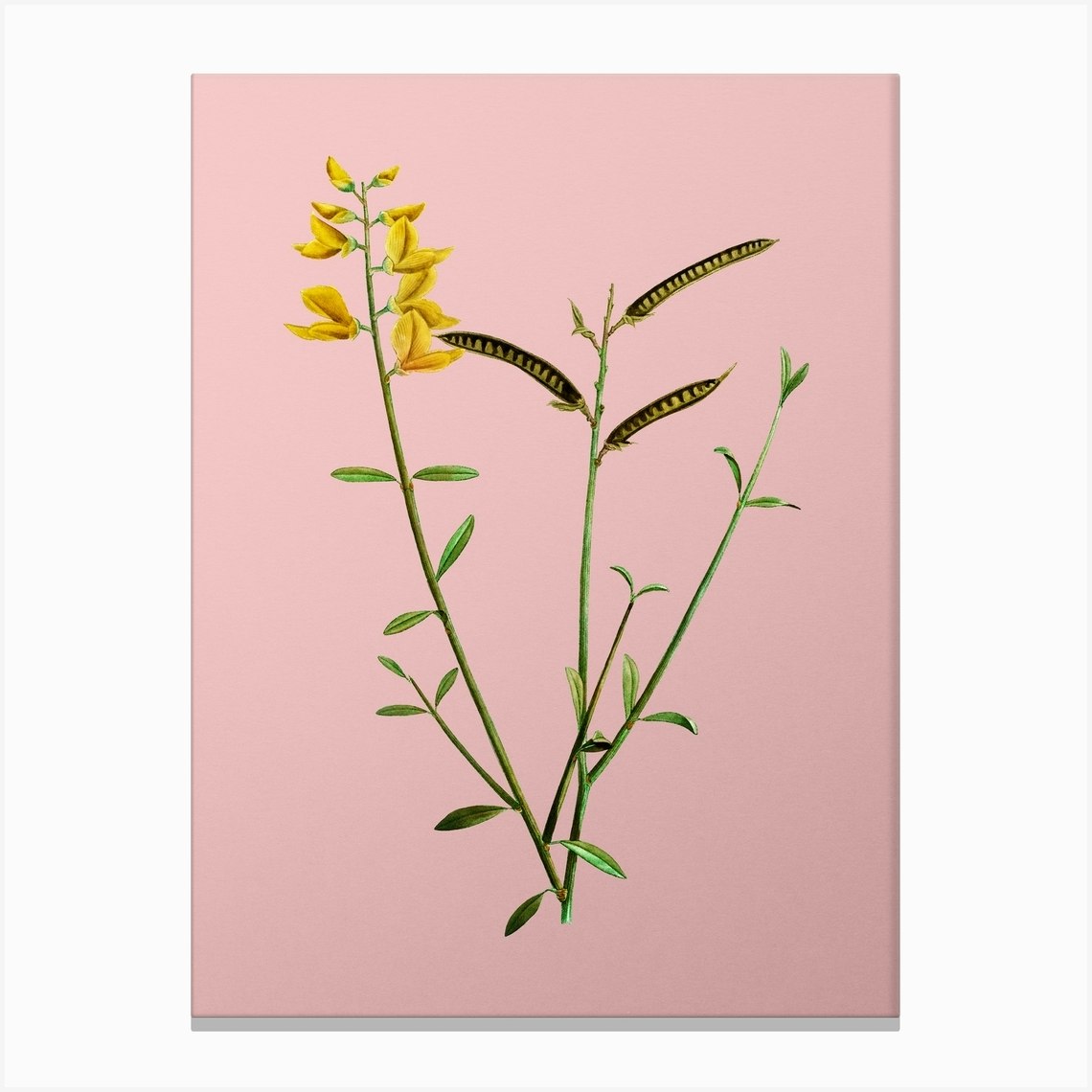The image is a detailed, simple illustration of a plant set against a light-pink, portrait-oriented background. The central plant consists of one main green stalk with four branches extending vertically. The largest branch, curving slightly to the left, features numerous narrow leaves and is topped with yellow flowers in varying stages of bloom. To the right of this main branch is another branch that has three brownish-yellow pea pod-like protrusions extending from it, arranged alternately. The two smaller branches on the far right are adorned solely with green leaves and do not bear any flowers or pods. The image is clearly an illustration, possibly a painting or drawing, and occupies the center of the pink background without any text or identifying markers. The overall color scheme includes the soft pink background, green leaves, yellow flowers, and brown pods.